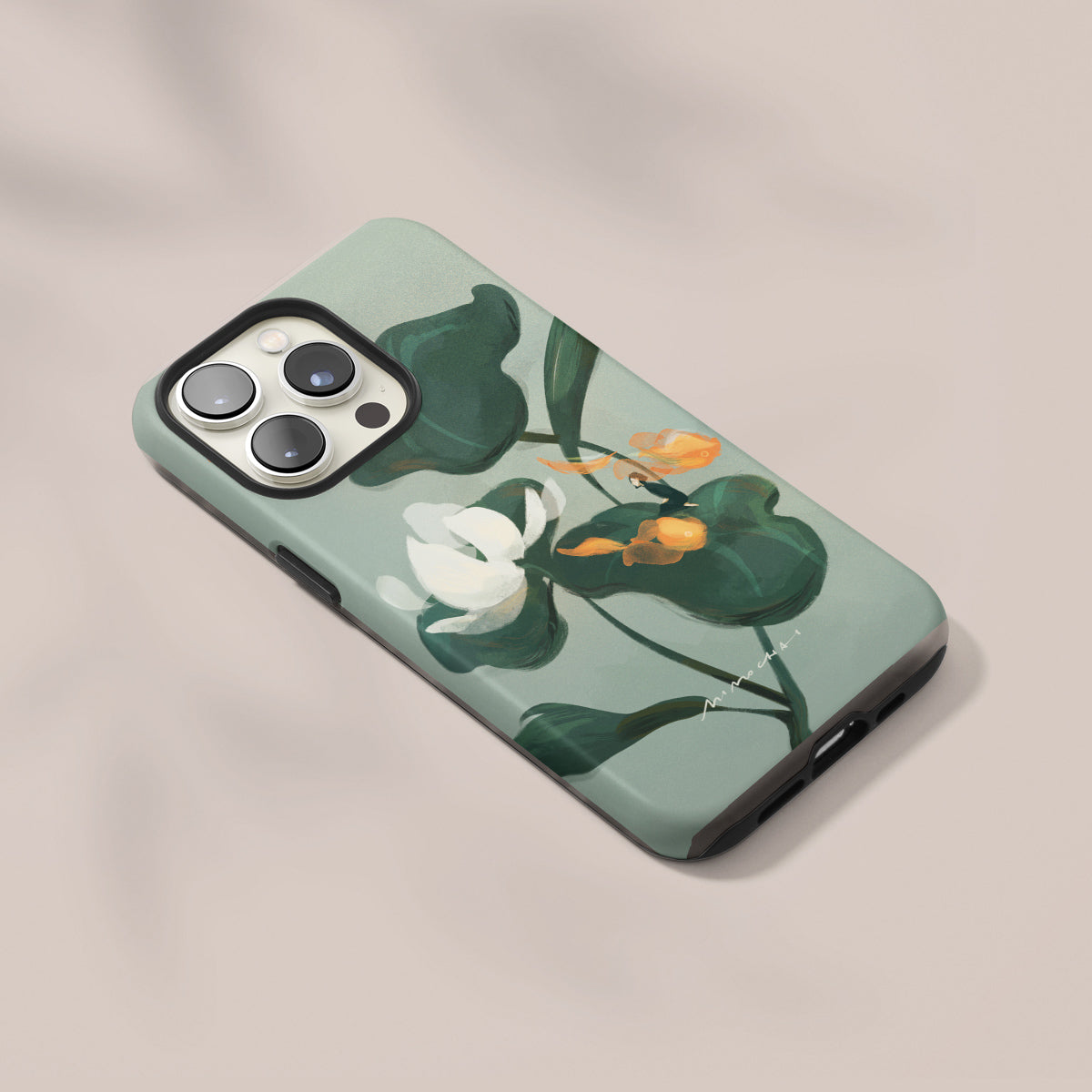The product photograph showcases a rectangular phone case designed for an iPhone, meticulously edited to be on a flat, light gray surface ideal for online commercial listings. The case, displayed face down on a white cell phone, reveals a detailed design: a light green background adorned with darker green leaves, reminiscent of a lily pond, and a white-petaled flower with hints of yellow. Adding to the whimsical nature, a small, delicately drawn miniature man sits on one of the leaves. The left upper corner of the phone frame features a square incision that accommodates the phone's three lenses. Contrasting the gentle green tones, the edges and bottom of the phone case are finished in black. The case's top and bottom edges are angled, with the top pointing towards the left and the bottom towards the right corner, enhancing the visual appeal of the product. The overall design appears hand-crafted and artistic, making it a charming, yet practical accessory for the device.